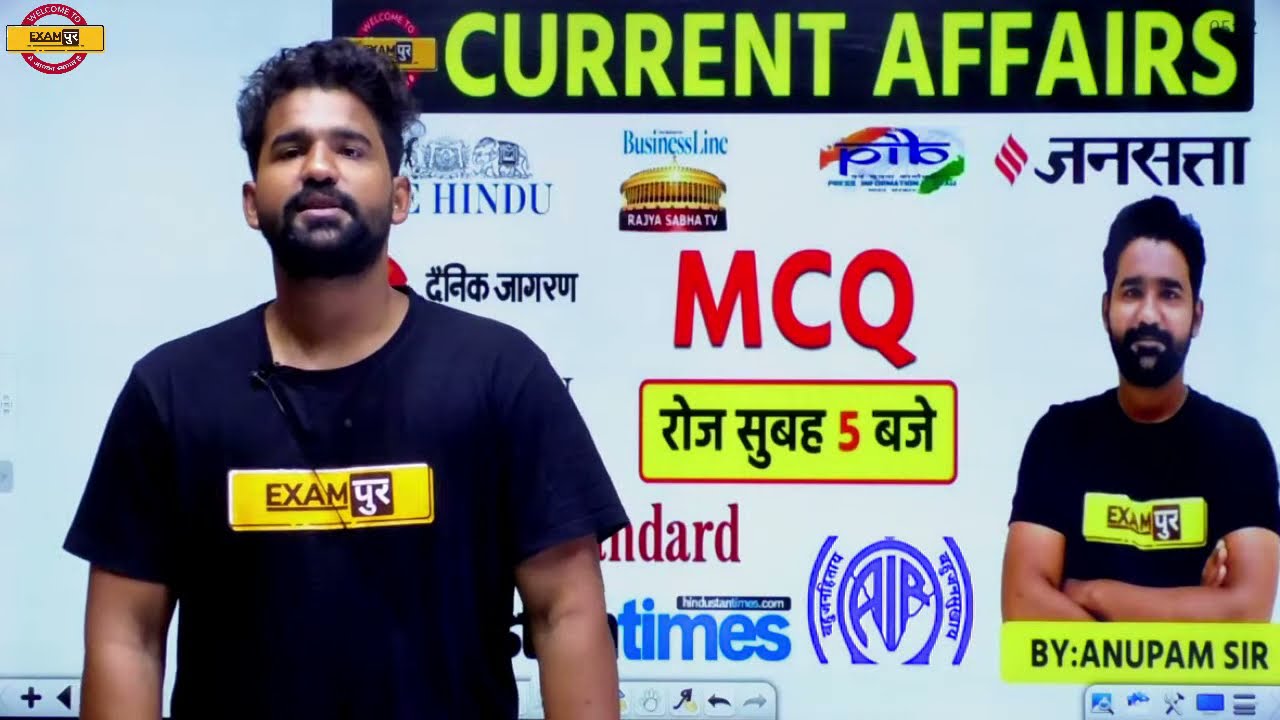The image showcases a young man standing on the left side, wearing a black short-sleeved t-shirt with a yellow rectangle on the chest that has the word "Exam" underlined in maroon text. The man, who has curly black hair, a black beard, and medium-tone skin, is also sporting a small black microphone clipped to his t-shirt. He appears to be in front of a backdrop filled with various logos and text, including "Current Affairs" in yellowish-green text at the top, and others like "Business Line," "Hindu," and "MCQ" in red, with additional symbols and text in a foreign language. There is also an image of the same man, looking skinnier, with his arms crossed, wearing the same t-shirt, and positioned on the right side of the backdrop. Below this image, there's a yellow bar with black text reading "by Anupam Sir." The overall scene suggests a screen grab from an online video stream, possibly of an educational web series focusing on current affairs.